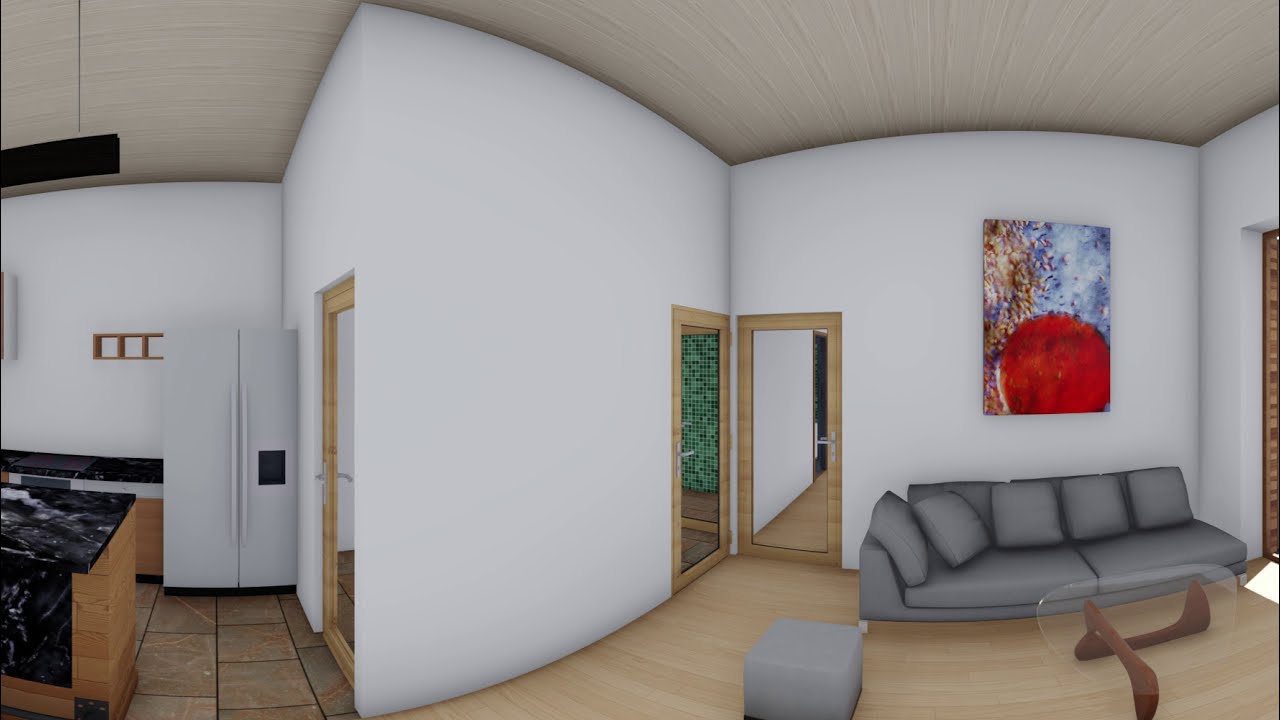This image is a detailed 360-degree panoramic screenshot from a simulation game, resembling a fisheye lens rendering of a modern, angular home's interior. The room features white walls and a light tan-gray ceiling, with light tan wood and beige tile flooring. On the left side, part of the kitchen is visible, showcasing a white double-doored refrigerator and black granite countertops with light tan wood accents. Adjacent to the kitchen is a mirrored door. Moving towards the center of the frame, two mirrored doors are positioned on opposite sides of a corner. To the right side of the image, a cozy living area boasts a gray couch, a matching gray ottoman, and a sleek glass-topped coffee table. Above the couch, a vibrant abstract painting with predominant red, blue, and yellow hues adds a splash of color to the scene. The room is unoccupied, emphasizing the architectural and design elements of this simulated house.